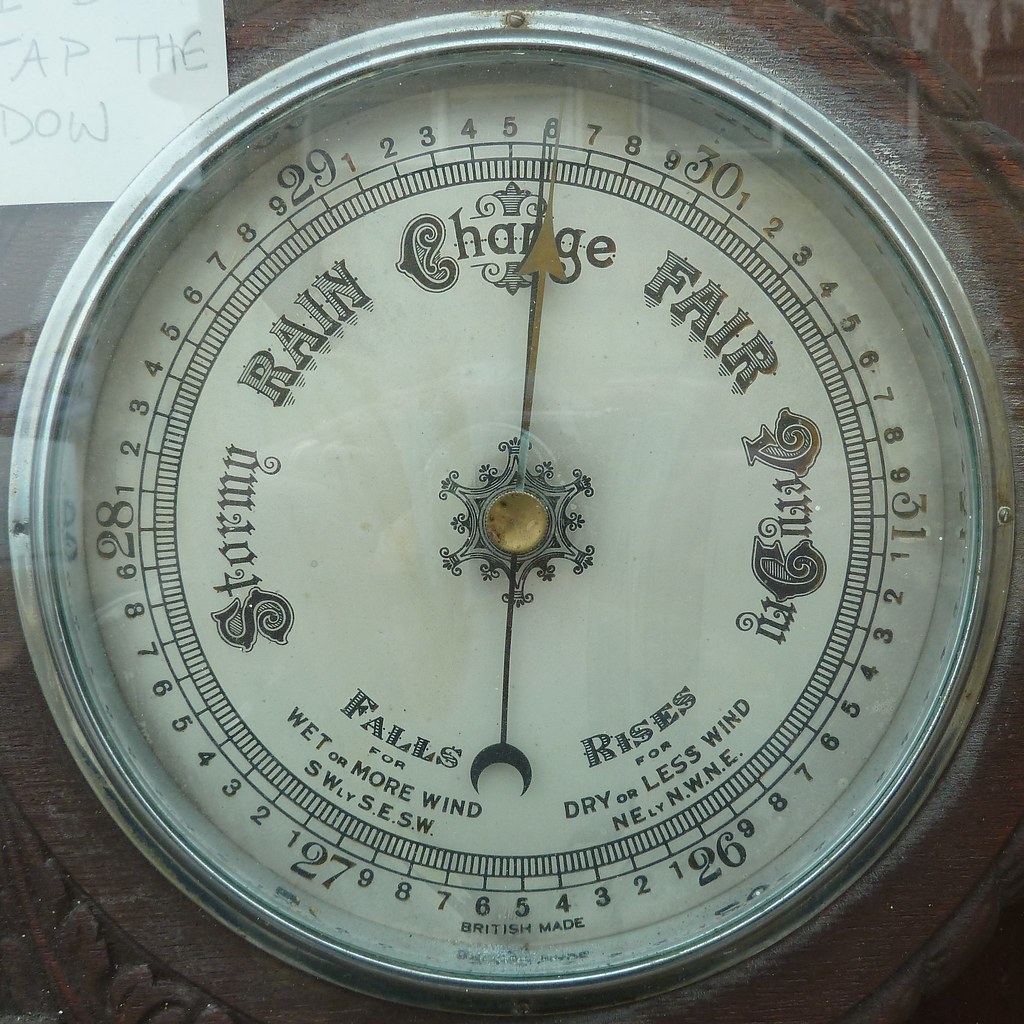The image depicts an antique barometer, likely made in Britain, which features a circular metal frame and a face marked with both large and small numbers. The large numbers, ranging from 26 to 31, frame the outer edge while smaller numbers from 1 to 9 repeat in sequence around the inner circle. At the center, a gold screw anchors two metal arrows—one a long metallic hand and the other a crescent moon-shaped pointer. 

The barometer’s face is also adorned with various weather-related notations such as "stormy," "rain," "change," "fair," "dry or less wind," and "wet or more wind." These annotations seem to align with likely wind directions, including northeast and southwest. The labels "29 to 31" and "1 through 9" indicate barometric pressures, reminiscent of a clock's layout, but designed to predict weather changes. The background appears to be wooden, suggesting it is attached to a dock or wall, emphasizing its rustic, historical charm.